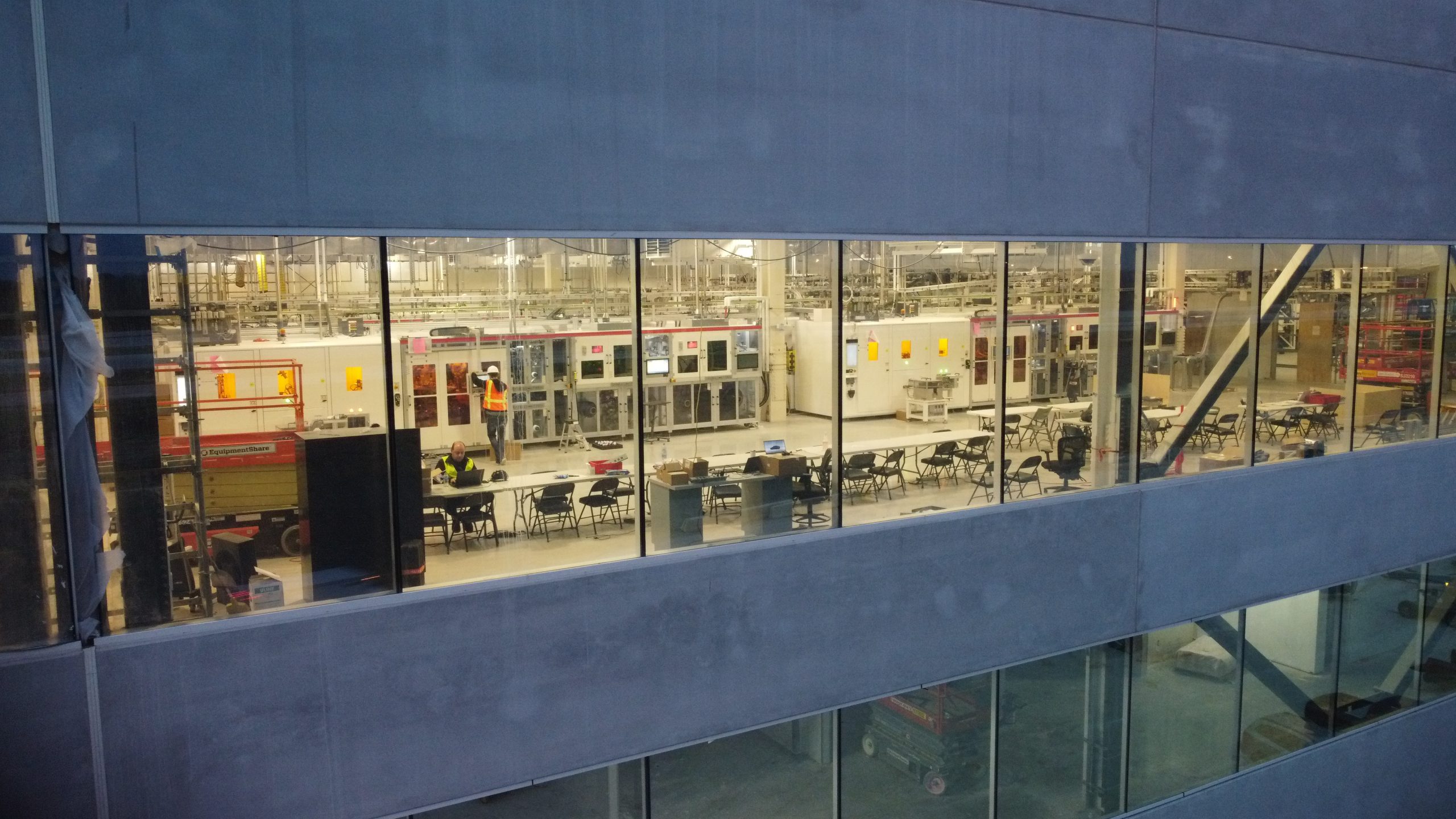The image depicts an industrial setting viewed from outside the windows of what appears to be a high-rise building, characterized by a wall of glass. Inside, a scene reminiscent of a manufacturing facility or factory unfolds. The interior features a row of plain white folding tables paired with dark blue and black folding chairs, where workers are seated, some wearing colorful safety vests. In the background, a display of various types of doors and cabinets stretches across, evocative of a Home Depot showcase. The space also contains warehouse equipment, such as a red scissor lift, and a worker is positioned near what appears to be a mechanical panel. The outer framework of the building consists of bluish-gray concrete or dulled metal, reinforcing the industrial aesthetic. The scene is a blend of functional office elements and heavy-duty manufacturing or warehouse apparatus.